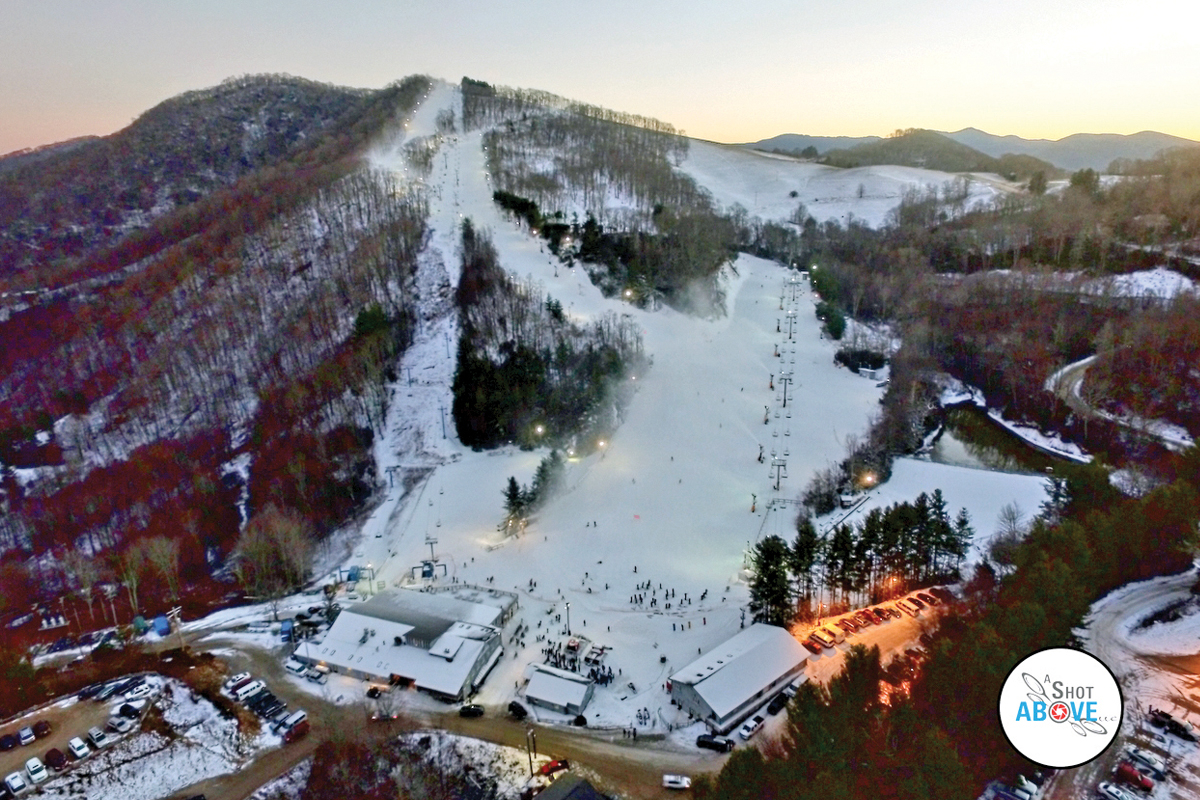This detailed aerial photograph captures a bustling ski resort nestled amidst snow-covered mountains. The light gray and white sky provides a subtle backdrop to the icy slopes that dominate the landscape. In the forefront, multiple brightly-lit parking areas are visible, with one particularly illuminated by yellow lights nearer to the center. Numerous cars fill these lots, hinting at the resort's popularity. The bottom left of the image reveals another parking space teeming with vehicles.

Prominent near the center-right, a ski lift stretches over the mountainous terrain, ferrying skiers to the snow-laden slopes. The slopes themselves promise thrilling runs for ski enthusiasts. At the base of the mountain, several buildings—large on the left, medium in the center, and small to the right—are blanketed in snow, with many people milling around, likely enjoying their winter escapade.

The photograph also features a distinct logo in the bottom right corner: a white circle with the text "shot above" embedded, where the letter 'O' is cleverly designed as a camera lens of a quadrotor drone, symbolizing the aerial perspective of the image. The combined elements of snowy peaks, lively resort activity, and detailed iconography create a vivid portrayal of a winter wonderland brimming with life and movement.